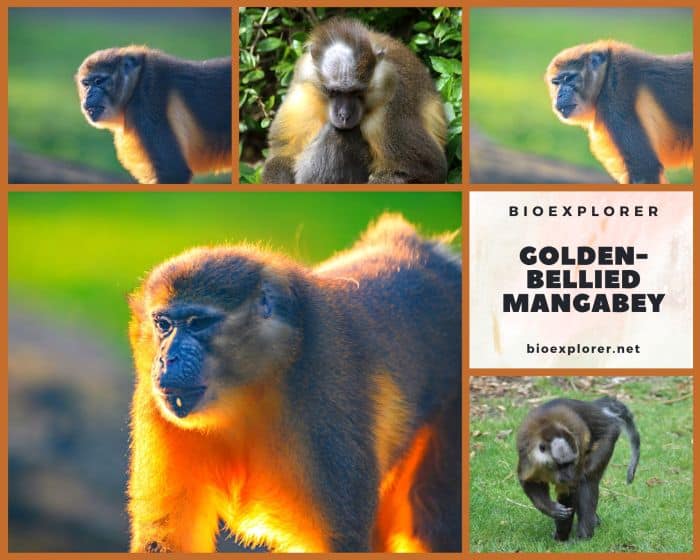The image is a high-definition collage comprising five photographs of a golden-bellied mangabey, set against a lush, forested backdrop with hints of hills and rocks, suggesting a daytime setting with sunlight illuminating the surroundings. Each photo is framed with a brown border, with one larger image occupying the lower left corner, while the others are of uniform size. This particular monkey, known for its distinctive golden fur around its belly, neck, and parts of its head which can appear orangish in some lighting, is highlighted in various poses throughout the mosaic. The center-right section of the collage features a white field with the title "bioexplorer golden-bellied mangabey" in bold black fonts, alongside the website bioexplorer.net.